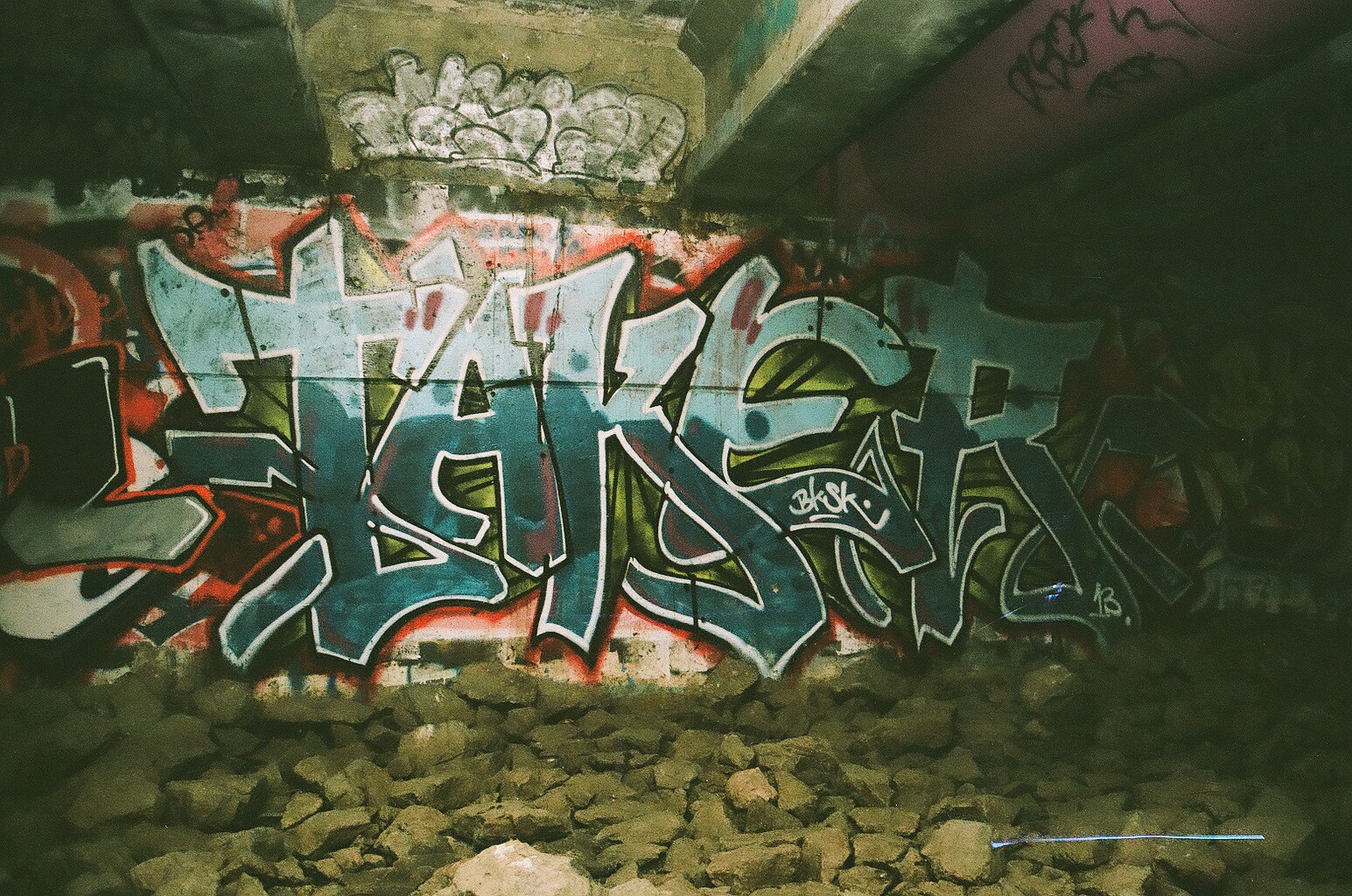The photograph features a dimly lit underground area, likely an underpass or tunnel, with a prominent concrete wall dominated by an elaborate piece of graffiti. The central graffiti, reading 'Taker' in stylized letters, transitions from dark greenish-blue at the bottom to light blue at the top, outlined in red, and backed by green spray paint. Surrounding this main word are additional tags and designs in black, red, and several other colors. Above the wall, on the surrounding structures, more graffiti in white is visible. The scene is illuminated only by the camera flash, highlighting the exposed ceiling beams and a large purple pipe on the right side of the frame. The ground in front of the wall is littered with loose, dirt-covered brown stones, contributing to the overall gritty and aged appearance of the setting.